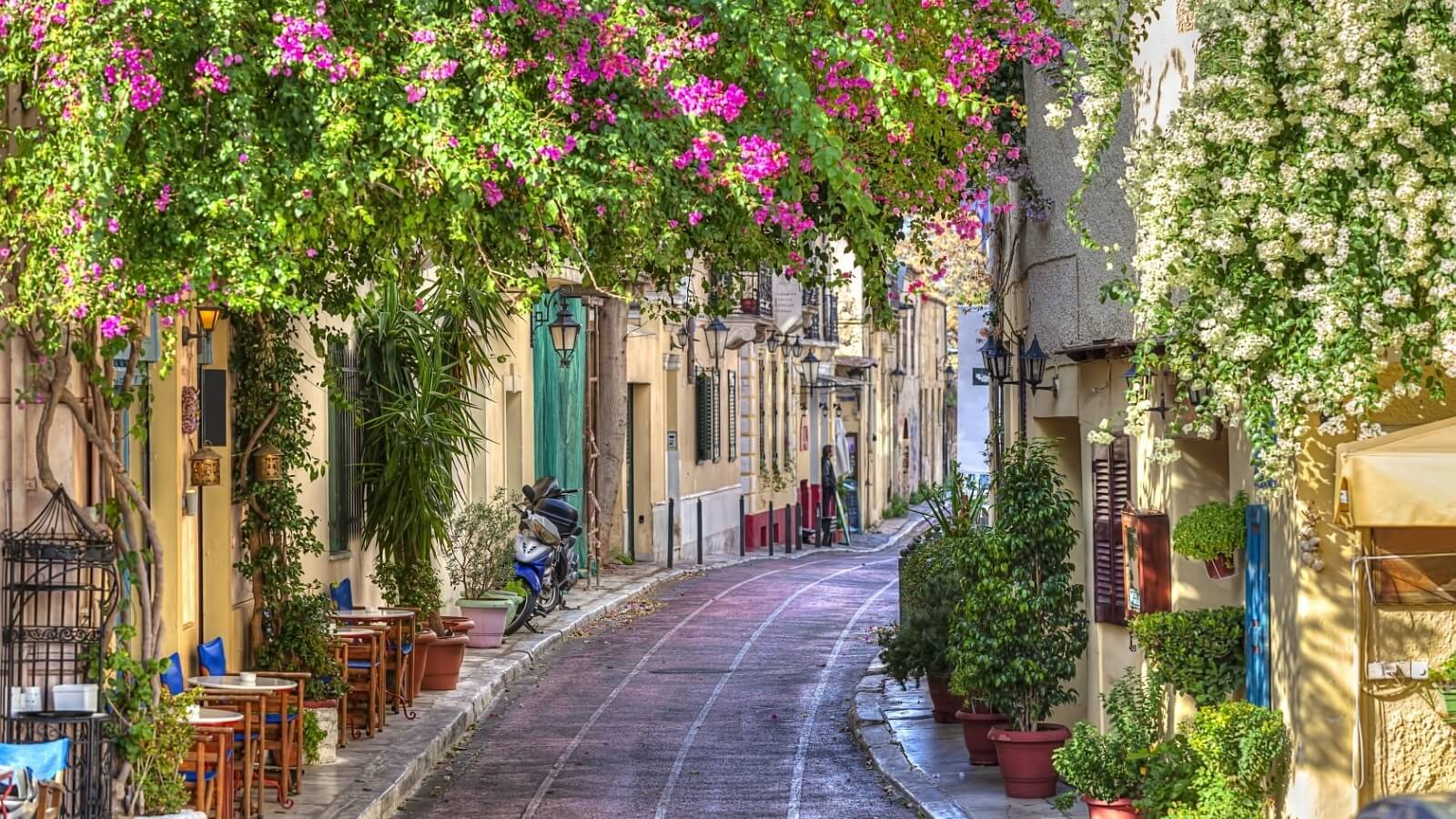This vibrant photograph captures a charming, narrow street, likely in a European city, possibly Italy. The street is bustling with lush greenery and vivid flowers, creating a beautiful overhang of predominantly pink bougainvillea mixed with some white blooms climbing the old, colorful buildings. The architecture speaks to an older, historical setting with walls painted in hues of yellow and light green, providing a picturesque backdrop. 

To the left, a quaint outdoor seating area with blue chairs and small tables is set up, hinting at a coffee shop or restaurant. On the cobblestone road, a sleek motorcycle is parked in front of an eye-catching green door, adding a dash of modernity to the rustic scene. A man in a black leather jacket stands nearby, perhaps waiting or admiring the lively ambiance. The sidewalk and street, though narrow, are teeming with life, adorned with various planters, vases with green shrubs, and trees. This idyllic streetscape, rich with colors and textures, exemplifies the elegance and charm of classic European city life.